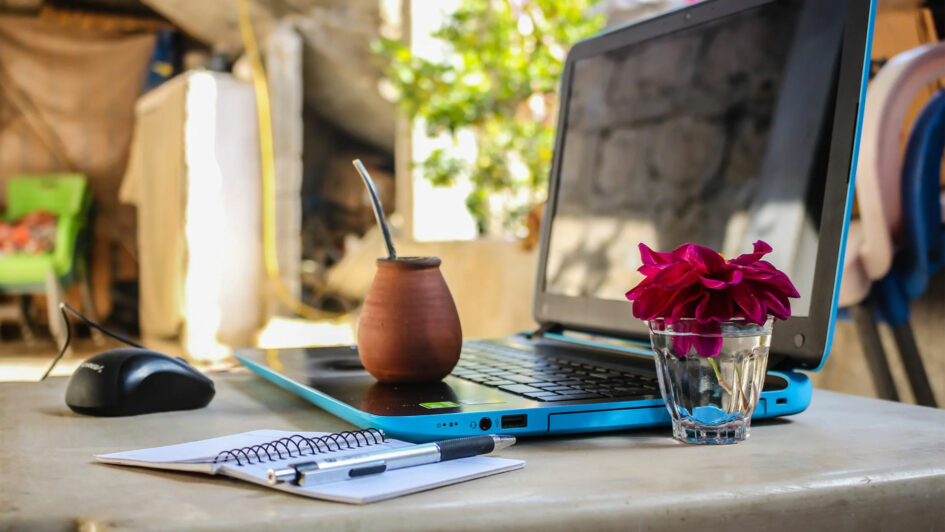The image depicts a close-up outdoor scene featuring a white marble table bathed in bright sunlight. The main focus is an open blue laptop, its screen reflecting the sunny environment with nothing visibly displayed. Resting on the trackpad of the laptop is a small wooden cup with a metal straw, suggesting it contains a drink. To the right of the laptop, there is a short glass of water with a single red flower and its stem submerged. In front of the laptop is an open notepad with white pages, on top of which lies a black ink pen. A black corded mouse is positioned to the left of the notepad. The background is slightly blurred but shows a tree and an open, sunlit area, giving the impression of being on a patio or in a backyard. Additional background details include a green stack of chairs on the left side and a blue chair with a white chair stacked on top of it on the right.